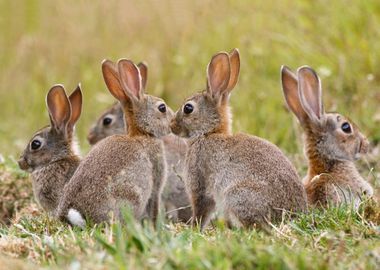In this detailed photograph, five brown bunny rabbits are gathered on a lush, green grassy terrain. Their pelts are a mix of light brown with hints of white and gray, giving them a soft, textured appearance. All five rabbits share common features: tall, flesh-toned pink ears that allow light to shine through, creating a glowing effect, and large, expressive black eyes encircled by delicate white rings.

At the foreground of the image, two of the bunnies, their small, white tails peeking out, are touching noses and facing each other with their backs turned to the camera. In the background, the other three rabbits are also facing away; the one on the right seems to be looking to the right, while the two on the left appear to be gazing to the left, indicating an intriguing interaction or alertness towards their surroundings. It's likely early morning or late evening, as the lighting suggests a soft, natural daylight scene with the light source coming from behind the camera. The overall composition offers a peaceful, scenic snapshot of these adorable creatures in their natural habitat.